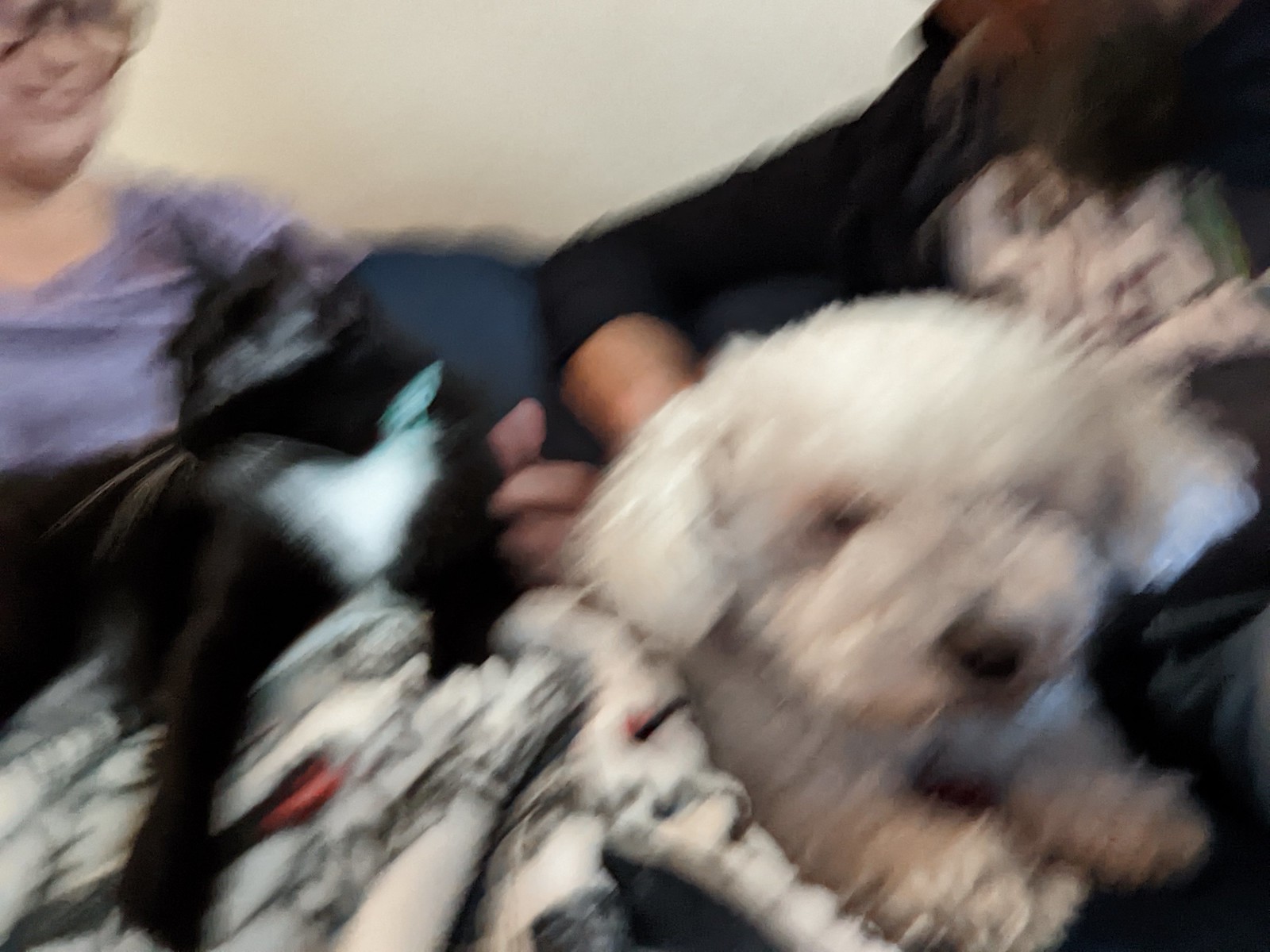In this rectangular and very blurry, low-resolution photograph, the main focus is on a couch positioned straight ahead. In the lower right corner, a white dog is prominently featured. It could either be a puppy or a smaller breed; its short-trimmed ears suggest a puppy-cut hairstyle. The dog has a button-black nose and similarly dark eyes, both adding to its distinct but fuzzy appearance. It is positioned directly on what seems to be a dark brown couch.

Above the dog, a tuxedo cat is also shown sitting forward with its paws extended outwards, although its gaze is directed to the left side of the image. Despite the blur, the cat’s black and white fur pattern is discernible, although its eyes are not visible.

In the upper left corner, a human figure is partially visible behind the cat. The person appears to be wearing a lavender or light blue scoop-neck shirt. Although the image is unclear, it is noticeable that the individual has white skin and is likely Caucasian, with a fragment of her eyeglasses faintly observable.